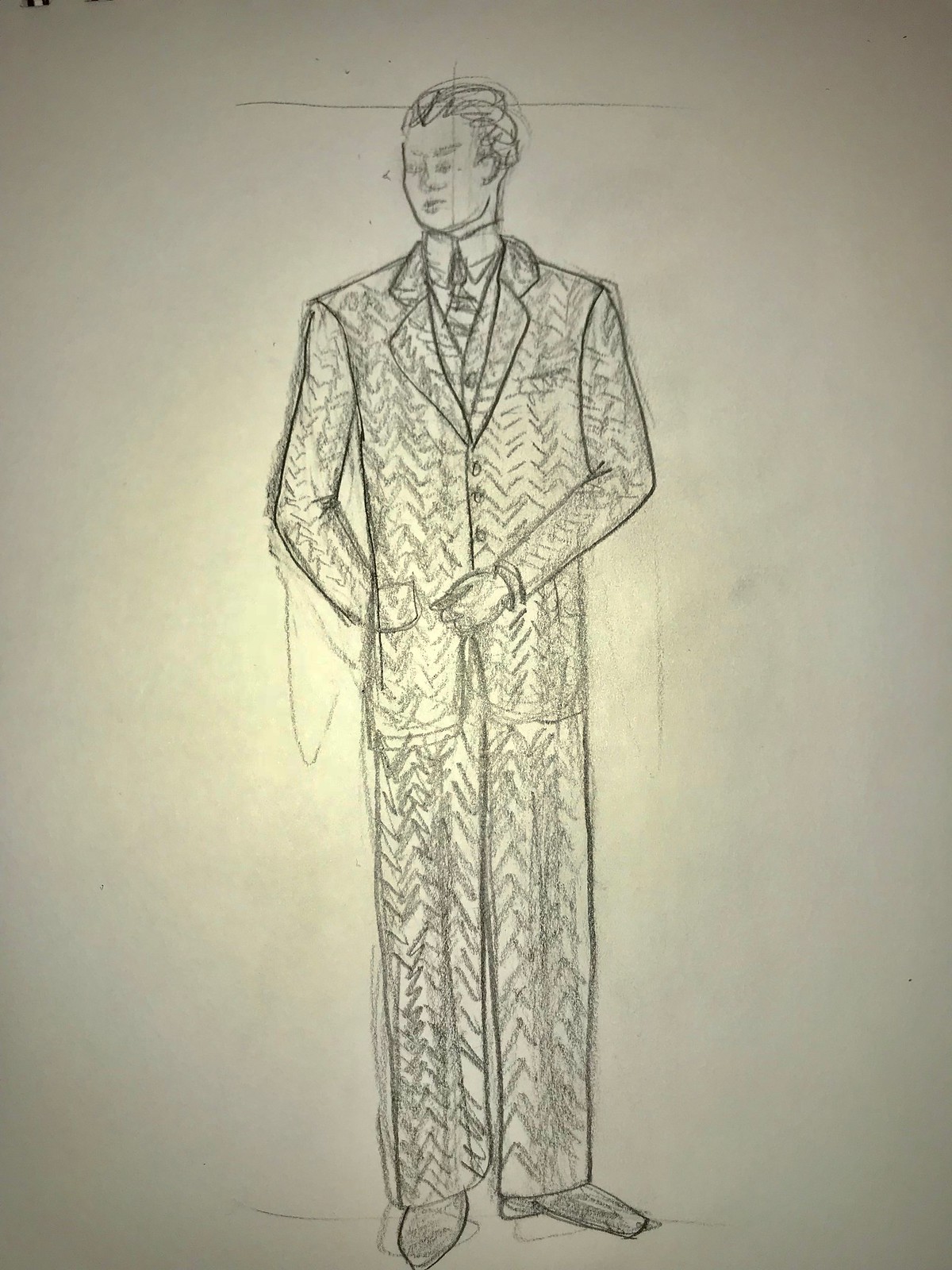This is a graphite pencil sketch of a man in a three-piece, single-breasted suit, possibly resembling tweed due to the textured shading. The man, who has short, neatly combed hair, is depicted with a collared shirt and a striped tie under his buttoned jacket. One of his hands is clenched into a fist and positioned in front of his stomach, while the other is folded behind his back, out of view. His shoes are black, and his slacks show a distinct crease, adding to the formal appearance. The man's facial features are vague, rendered with simple shading and contour lines. The sketch shows evidence of rough guides with horizontal and vertical lines over the head, likely used during the initial stages of drawing. In the top left corner of the white paper, there are two holes and black lines that suggest it was part of a spiral notebook. The photograph of the sketch has darker edges and a brighter center, likely taken with a flash, and exhibits signs of erased marks, indicating multiple attempts by the artist.